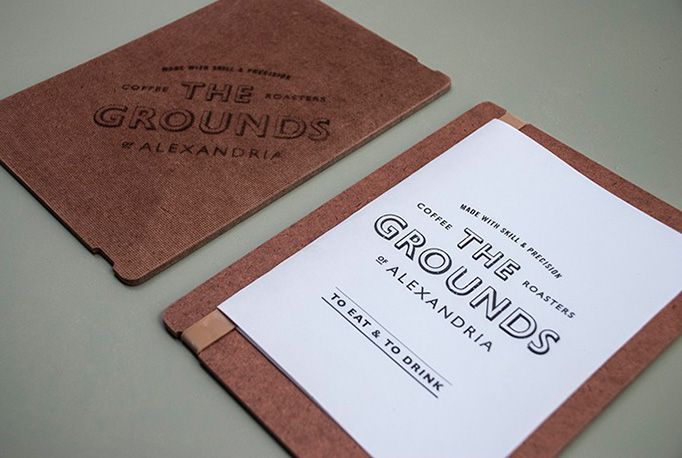The image features two menu-like objects positioned side by side on a white background that resembles a table. Each menu is bound in a textured, leather-like material. The left menu is closed, showcasing the cover which reads "The Grounds Alexandria," indicating it belongs to a coffee roaster shop called The Grounds in Alexandria. The right menu is open, with its first page displaying the text "Made with skill and precision, The Grounds Coffee Roasters of Alexandria. To eat and to drink." This suggests a focus on both food and beverages, typical of a specialty coffee shop. The colors presented are the white of the menu pages, the brown leather binding, and a tan background, giving the composition a cozy, artisanal feel. Both menus are slightly tilted and placed in such a way that they create a balanced arrangement. The overall scene conveys the aesthetic and branding of an independent, possibly specialty coffee shop.